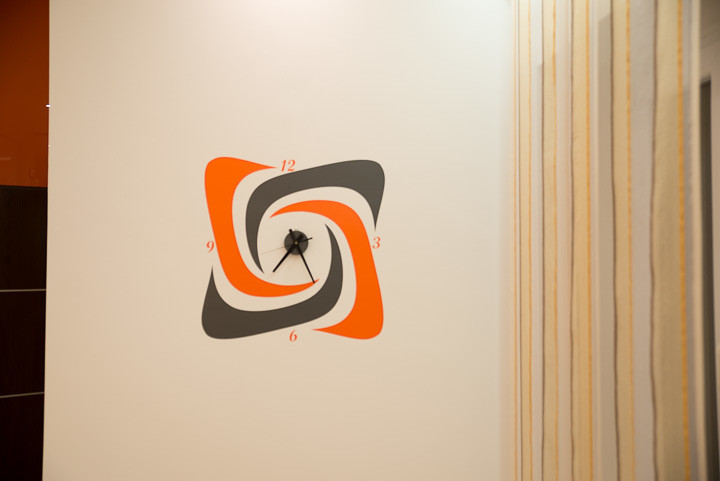This photograph features a uniquely designed wall clock that almost appears to be integrated into the wall itself, devoid of a conventional housing or visible frame. The centerpiece of the clock is a black circular dial with three black hands—an hour hand, a minute hand, and a second hand—indicating the time. Surrounding the clock are four distinct swirl patterns in forms resembling a stylized 'C,' painted in alternating colors of orange and gray. These swirls radiate from the center and align with the numbers 12, 3, 6, and 9, which are situated at their respective positions on the dial. The uppermost swirl at the 12 is orange; the next, located by the 3, is gray; the one by the 6 is orange; and the last, near the 9, is gray. The entire design evokes a sense of dynamism and an artistic flair, as though the clock and its swirling embellishments are seamlessly integrated into the wall, creating an almost surreal timepiece. Surrounding the clock pattern, the wall itself has additional design elements, including a thin burgundy red border on the left and a section of black rectangles just below it. A hint of an open doorway and various colored borders—orange, yellow, and gray—add further complexity and color to the composition, enhancing its abstract and unconventional aesthetic.